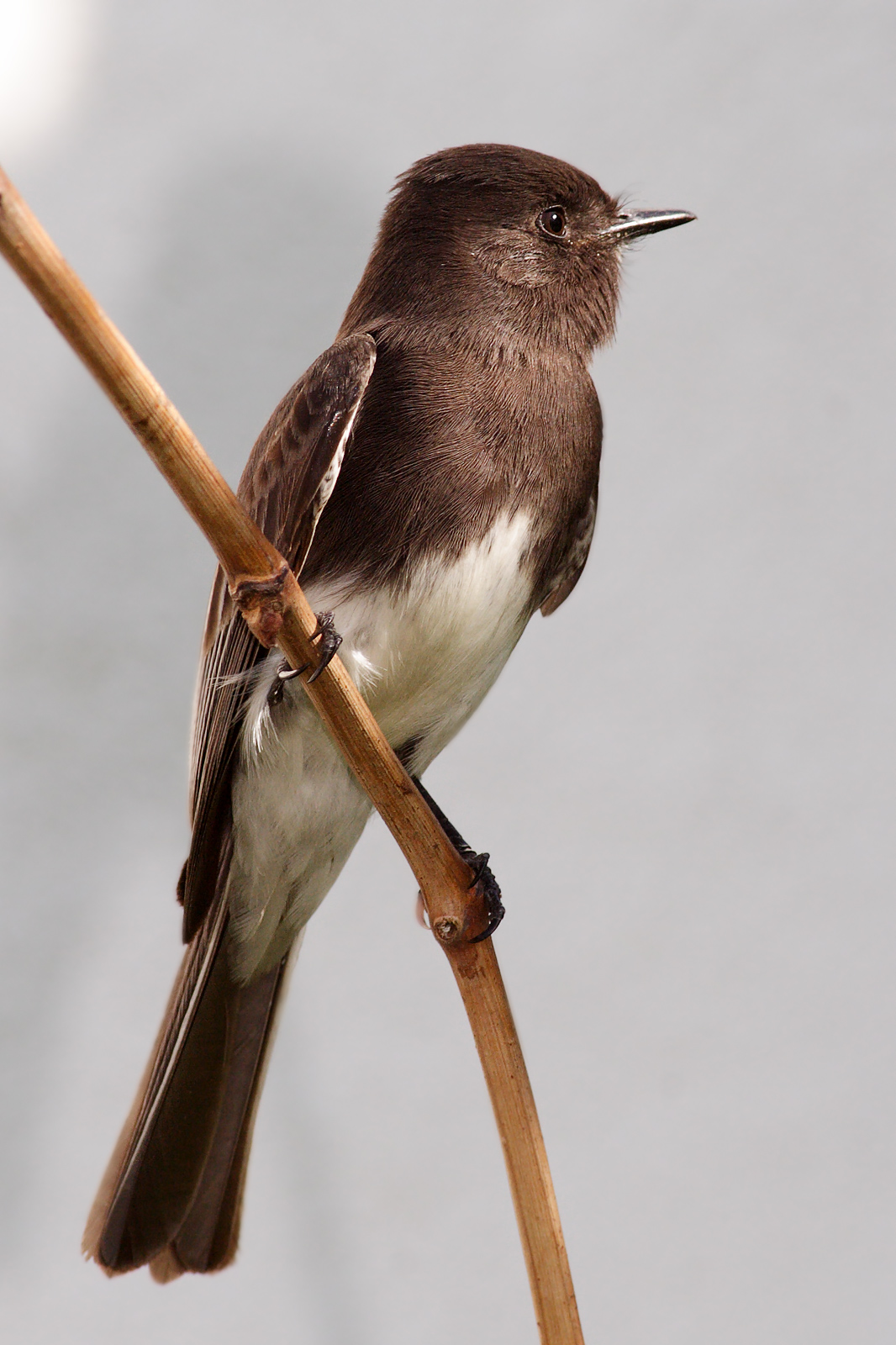This vertically oriented bird portrait features a medium-sized bird perched prominently on a light brown, stripped branch against a flat gray background. The bird's dark brown talons grip the thin branch securely. Its head aligns closely with its body, positioned centrally in the image. Its tail points slightly diagonally towards the lower left-hand side.

The bird boasts beautiful dark brown plumage and exhibits a short, thin beak colored black or gray. The bird’s head, tilted to the left, gazes towards the upper right corner of the frame. Its feathers appear sleek and smooth against its head and white underbelly, while its side wings rest tightly against its body. The wings display a rich mix of dark and light brown hues with varied textures, creating a mottled effect. Notably, the tip of the tail appears slightly blurry, suggesting motion or a depth of field effect. This detailed and vibrant portrait captures the bird with an almost artistic precision, possibly enhanced through a design program to accentuate its natural beauty.